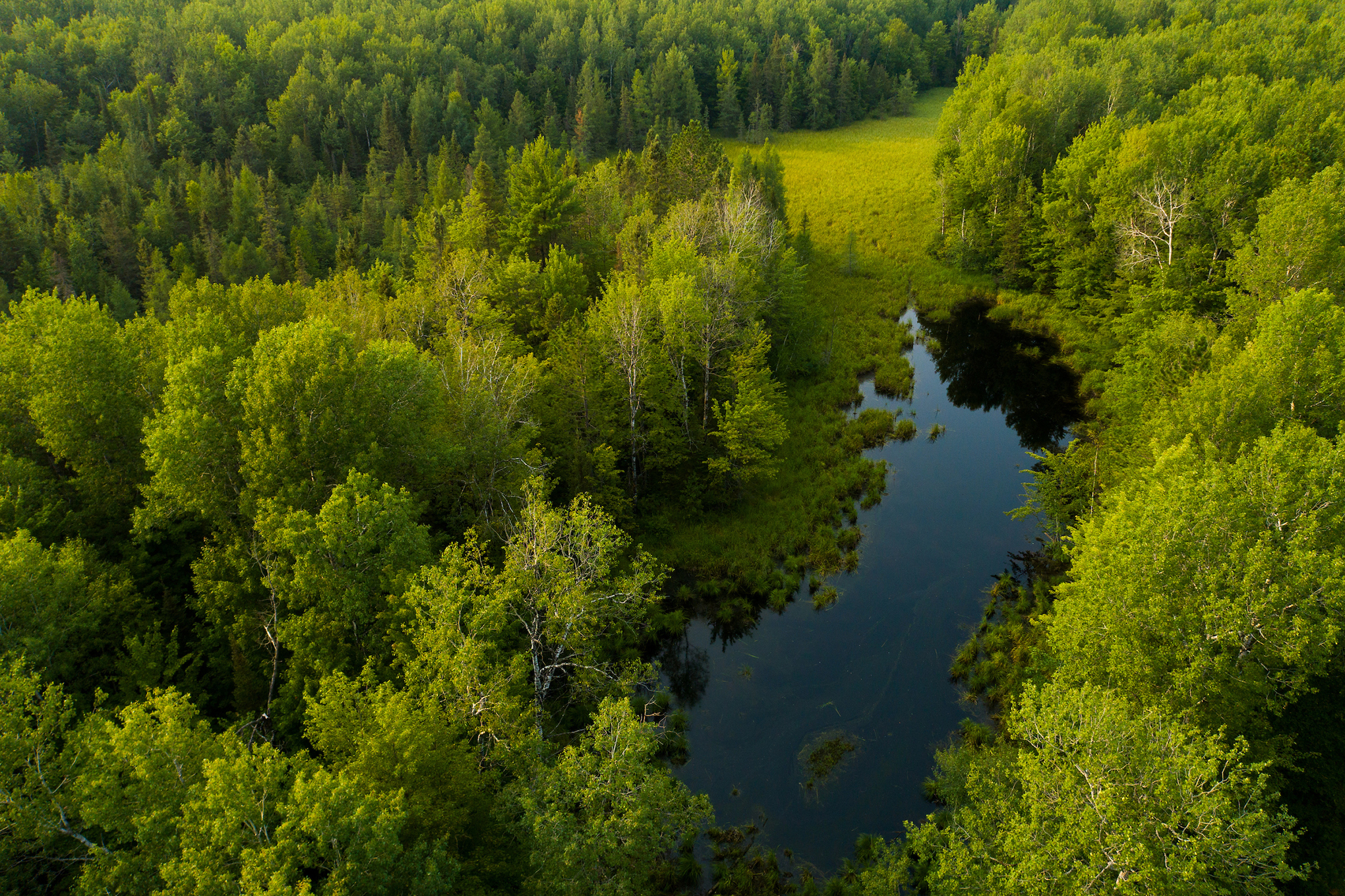The image showcases an aerial view of a nature area featuring a diverse landscape. Dominating the scene is an expansive forest with a mix of light and dark green foliage, interspersed with occasional splashes of orange and white from the branches. At the heart of this verdant tapestry lies a small pond, its waters reflecting varying hues of blue, from light to dark. The pond is situated slightly to the right of the center and is surrounded by the dense forest. Above the pond, an open meadow of light green grass extends, providing a fresh contrast to the surrounding woods. The image captures a peaceful and serene environment, highlighting the harmonious coexistence of open grassy meadows, a tranquil pond, and a lush forest teeming with trees.